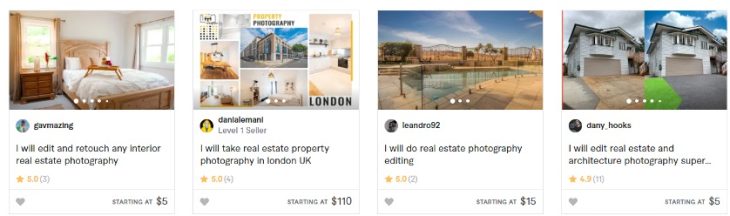This landscape-mode screenshot, likely taken from a website viewed on a laptop, displays a page featuring four distinct columns. Each column showcases a service offered by different individuals related to real estate and property photography.

1. **First Column:**
   - **Visual:** The photograph captures a cozy bedroom boasting two large windows that offer a view outside. The neatly made bed features a breakfast tray, enhancing the inviting ambiance.
   - **Description:** "Gavmazing: I will edit and retouch any interior real estate photography."
   - **Ratings and Pricing:** The service has a rating of five stars and starts at $5.

2. **Second Column:**
   - **Visual:** A collection of images depicting various buildings, indicating expertise in property photography.
   - **Description:** "Danielle Mani: Level One Seller. I will take real estate property photography in London, UK."
   - **Ratings and Pricing:** This service is also rated with five stars and starts at $110.

3. **Third Column:**
   - **Visual:** A vibrant landscape photo characterized by a desert-like environment under a bright blue sky.
   - **Description:** "Leandro92: I will do real estate photography editing."
   - **Ratings and Pricing:** The service is priced starting at $15.

4. **Fourth Column:**
   - **Visual:** A comparison image showing two columns; the first displays the original photo, while the second shows enhancements such as a bluer sky, better driveway, and improved grass.
   - **Description:** "Danny Hooks: I will edit real estate and architecture photography super."
   - **Ratings and Pricing:** This service also has a starting price of $5.

The website appears to be a freelancing platform where users list their services and specify their starting rates and reviews.